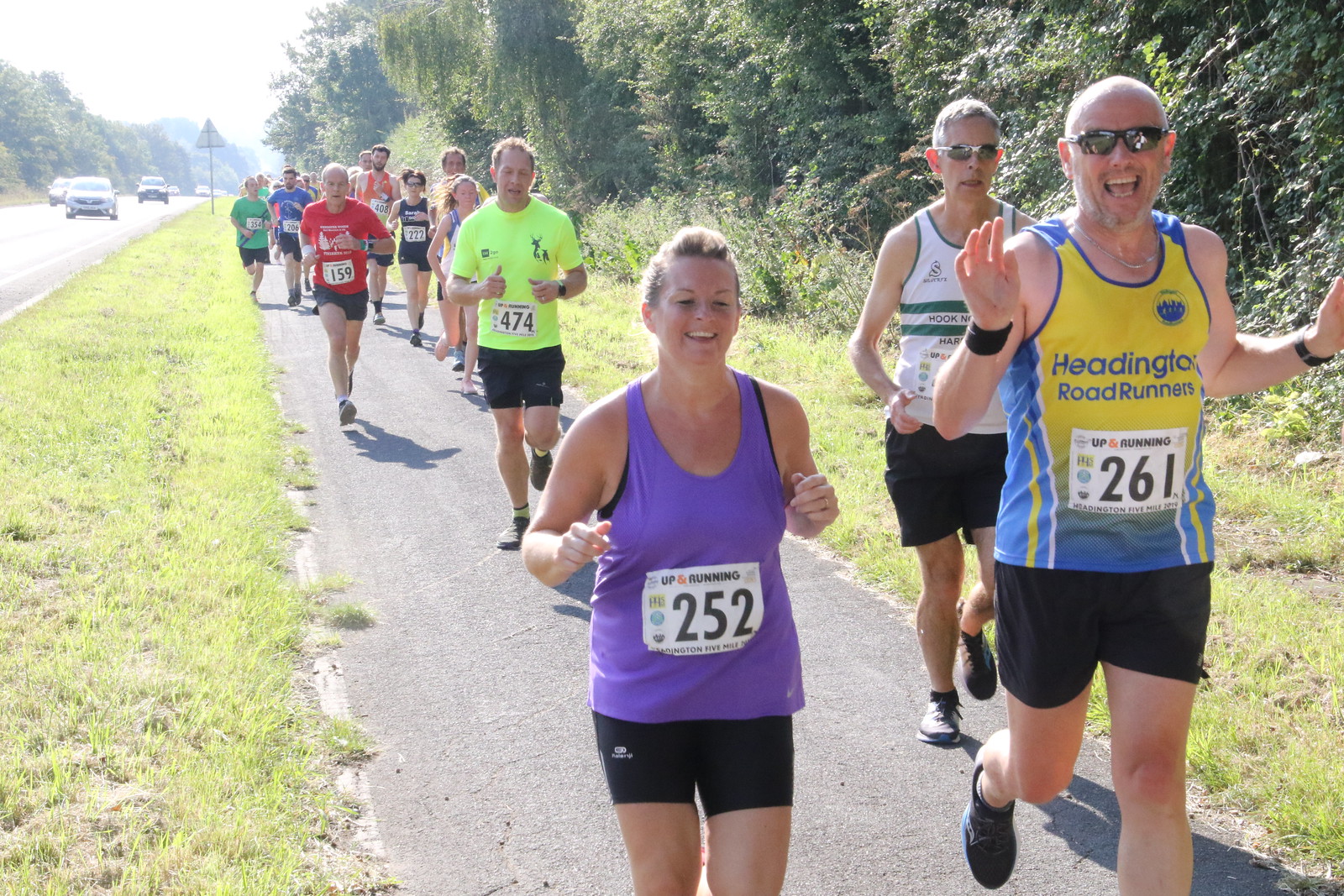In the image, a bustling marathon is taking place along a paved sidewalk flanked by green grass and trees under a sunny sky, indicating a summer setting. On the opposite side of the path, a highway filled with fast-moving cars runs parallel. Numerous runners, all sporting numbered bibs on their fronts, dominate the scene. Prominently, a focused woman with number 251 and a cheerful man with number 261, his hands raised in a wave, are running in the foreground. Other identifiable runners include number 474 in a lime green shirt and number 159 in a red shirt. The runners in the lead wear tank tops—one purple, another yellow and blue—while everyone is dressed in shorts, embodying an active and vibrant atmosphere.